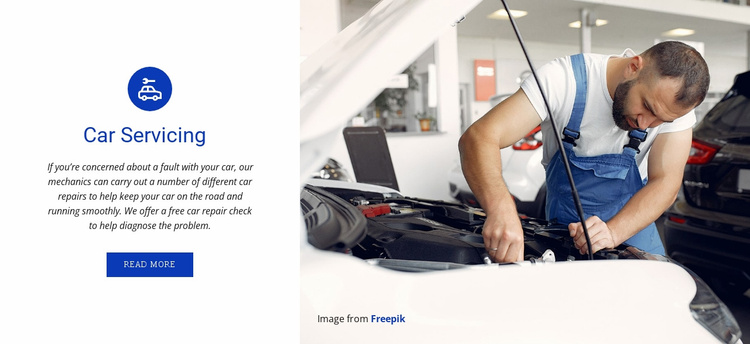**Detailed Caption:**

The image captures an auto repair scene with a focus on a mechanic performing maintenance on a vehicle. To the left, a prominent blue circle icon displays a car and a wrench, accompanied by the text: "If you're concerned about a fault with your car, our mechanics can carry out a number of different car repairs to help keep your car on the road and running smoothly. We offer a free car repair check to help diagnose the problem." A blue "Read More" button is also visible. 

In the foreground, a man dressed in a white t-shirt and blue overalls works diligently under the hood of a white car, which is held up by a black stick. The man has short dark hair, a mustache, a beard, and wears a wedding ring. Behind the white car, a black vehicle is parked. To the left of the scene, inside the repair shop, an office area is visible. The office features a window for customer transactions, a cup holder with pens, and recessed lighting. The interior of the building is painted white, providing a clean and professional appearance. This image, sourced from Freepick, illustrates a diligent mechanic ensuring a car is in optimal condition, with the backdrop of a busy automotive repair environment.